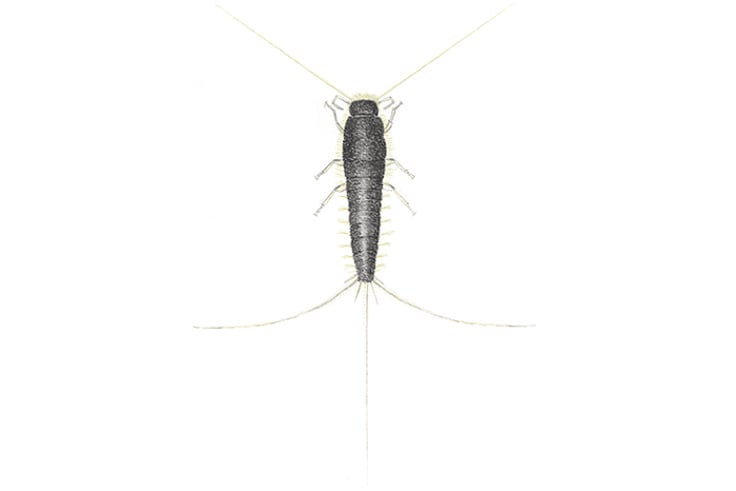This detailed illustration depicts a long, cylindrical water bug with a segmented black body and yellow, almost translucent limbs and antennae. The image, appearing as a black and yellow sketch rather than a photograph, portrays the bug with six primary legs—front, mid, and hind. The bug features two long antennae extending diagonally to the left and right from its head, which also has two shorter antennae. Near the bug's tail, three additional long tendrils are visible: one extending straight back and two curving to the left and right. Each of the approximately ten body segments includes pairs of small yellow furs protruding laterally. The bug lies stationary, flat on the surface, its meticulous details emphasizing the precision of the illustration.